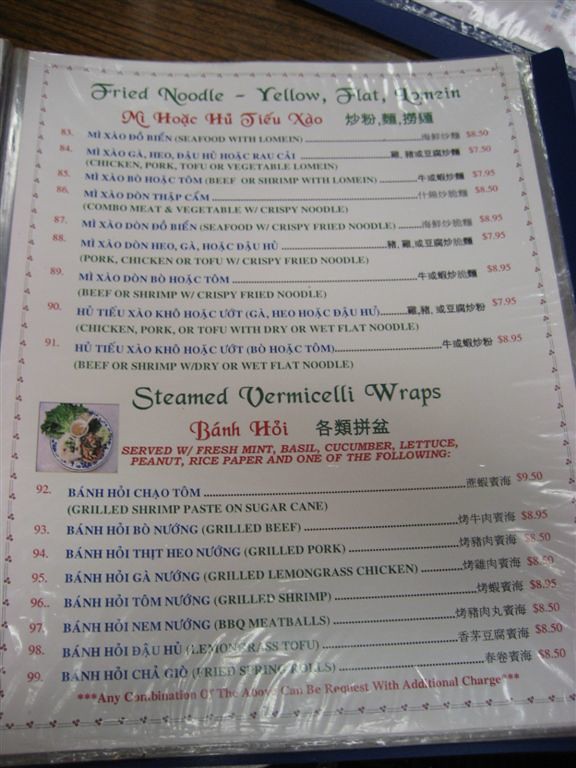This image depicts a Chinese takeout menu, meticulously wrapped in plastic. The majority of the text is in Chinese, with some English translations interspersed. The English descriptions start with "fried noodle" and "yellow, black," among other dishes. A specific entry details "Seafood with Lo Mein" priced at $8.50.

Beneath the Chinese text, printed in blue, are English descriptions in green. These include various Lo Mein options such as chicken, pork, tofu, or vegetable; beef or shrimp; and combinations like chop suey, which comprises a mix of meat and vegetables with crispy noodles. Other entries feature seafood with crispy noodles and pork, chicken, or tofu with crisp fried noodles. More options include beef or shrimp with fried noodles and combinations of wet or dry flat noodles with chicken, pork, tofu, beef, or shrimp.

Another section of the menu highlights "Steamed Vermicelli Wraps," served with fresh mint, basil, cucumber, lettuce, peanuts, rice paper, and a choice of grilled shrimp paste on sugar cane, grilled beef, grilled pork, grilled lemongrass chicken, grilled shrimp, barbecue meatballs, lemongrass tofu, or fried spring rolls.

Accompanying the text are images, including one that appears to show egg drop soup, a small container of soy sauce, lo mein, and a large lettuce leaf. The menu is decorated with intricate borders, adding a touch of elegance to its presentation.